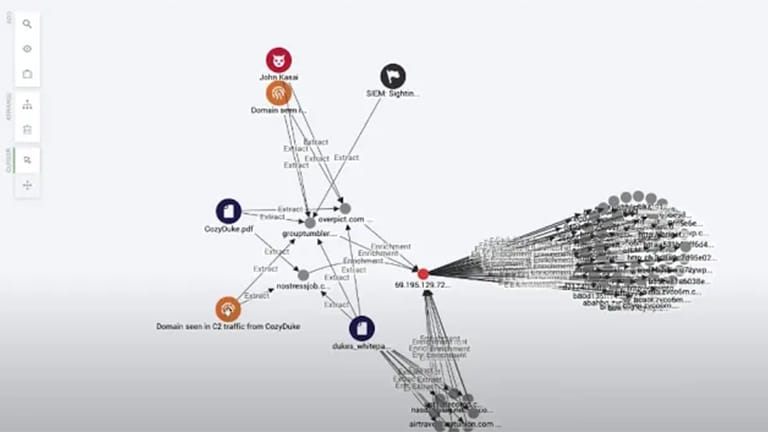The image appears to be a digital diagram set against a white background. It prominently features various colored circles, each containing different icons. At the top, there is a large red circle with the face of a cat in its center and the name "John Cassie" displayed below it. This circle is connected by black lines and arrows to other circles scattered around the diagram. These connections form a network of sorts, suggesting the tracking or flow of information.

There are additional circles with varying icons: an orange circle with a fingerprint, a blue circle with a piece of paper, and multiple black circles, one of which contains a flag. Black arrows point between these circles, indicating directionality or a sequence. On the left-hand side, there is what seems to be a drop-down menu icon, featuring symbols like a magnifying glass and an eye, further suggesting a digital or interactive nature.

In the top corners, there are dots, including a black dot with a flag and lines with arrows pointing towards it, adding to the detailed network structure. The overall aesthetic is quite schematic and precise, indicative of a technological or instructional chart.